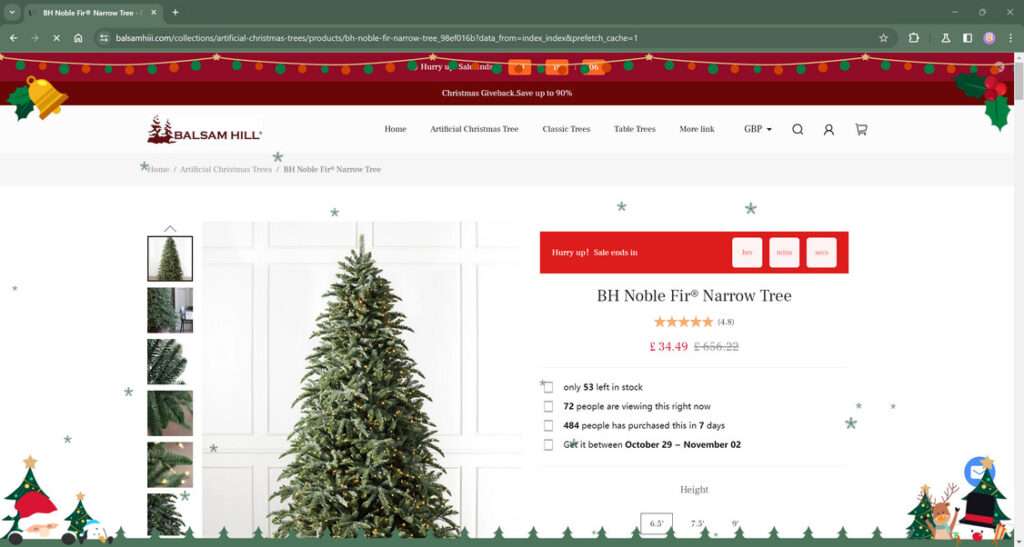**Screenshot Description: Balsam Hill Christmas Tree Sale Page**

This image is a screenshot of a webpage from a business specializing in Christmas trees. At the very top, there is a banner featuring "BH Noble Fir" and a mention of "Balsam Tree," although the text is somewhat blurry and difficult to read clearly. Below this, another banner with alternating red and green balls runs across the screen, culminating in a yellow bell with green leaves on the left and an image of mistletoe on the right.

The main body of the page is set against a stark white background with a notable burgundy text stating "Balsam Hill" alongside a Christmas tree icon. A series of navigation tabs are visible, including options such as "Home," "Two Streets," and "Table Trees."

Prominently displayed is an image of a Balsam Fir tree. The tree is described as being narrow at the top and full at the bottom, showcasing a lush green appearance. Adjacent to this, labeled as the "BH Noble Fir Narrow Tree," the product has an impressive rating of 4.9 stars. The price is listed at £34.49.

Below the price, a box provides additional details, including check boxes for ordering. Information highlighted in this section includes: "Only 53 left," "74 people viewing this right now," and "484 people purchased this in the last 7 days." Delivery is available between October 29th and November 2nd.